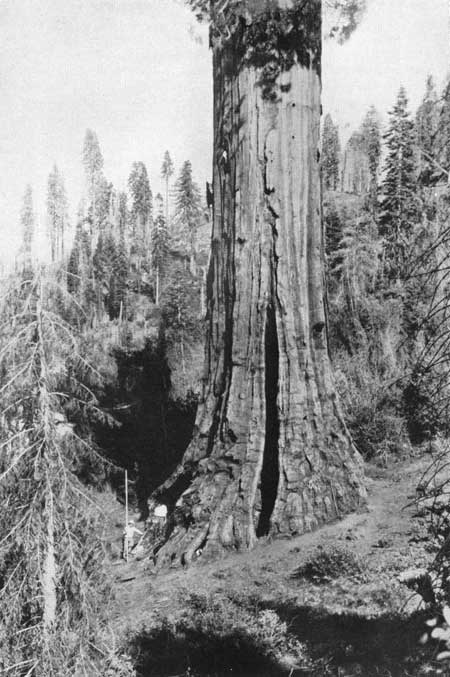This is a black and white daytime photo capturing a large red oak tree, prominently positioned at the center of the frame. The image is zoomed-in, highlighting a significant portion of the tree trunk with a visible crack that starts at the base and extends upwards for approximately 20 feet. The tree is uniquely growing on a slant, pitched downward, and surrounded by patches of grass and bushes at its base. Although the top of the oak tree is not fully visible, some foliage from its crown is discernible at the top of the photo. The background reveals numerous single pine trees and patches of open dirt, all bathed in natural light. The sunlight is coming from the side of the photographer, casting the oak tree's shadow onto the surrounding flora. The photo, devoid of any text or numbers, clearly focuses on the giant oak within a wooded, natural setting. The overall tonal palette varies from deep blacks to light grays, enhancing the sharpness and clarity of the scene.